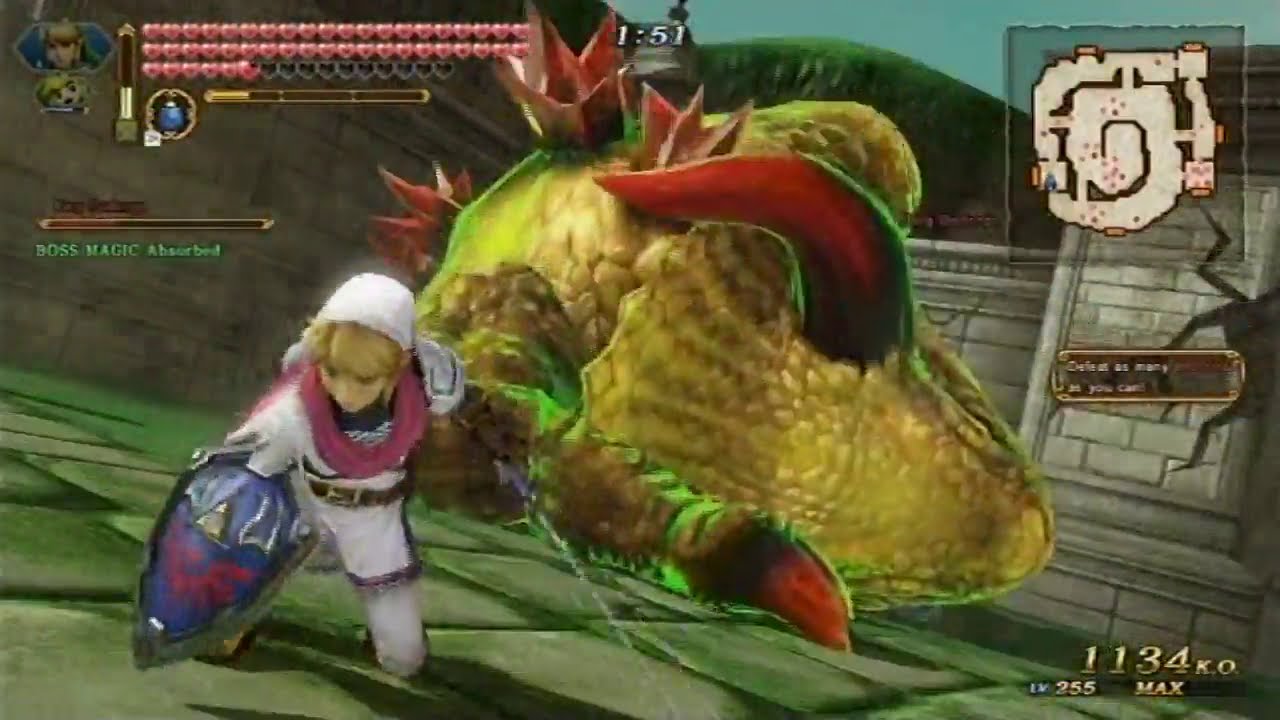The image is a screenshot from a fantasy video game, likely resembling "The Legend of Zelda." Dominating the foreground is the main character, potentially Link, who has blonde hair and is dressed in a white uniform with black trim, a dark pink scarf, and a white hood or hat. Equipped for battle, the character wields a blue shield in the right hand and a sword in the left hand, also wearing a glove.

In the background, a large, defeated creature lies on the ground. This monster is strikingly large, with a form that resembles an anatomical heart, primarily yellow with hints of green and brown, and adorned with red, tentacle-like appendages or possibly large red horns. The creature's size notably dwarfs the character and suggests a recent intense battle.

The setting appears to be an ancient, overgrown temple or a castle-like environment, featuring rugged bricks and possibly some paved stones, amidst a green landscape. The Heads-Up Display (HUD) is visible around the borders of the screen, showing elements such as a heart-based health indicator in the top-left corner, a map in the top-right corner, and various stats and text in the bottom-right corner that read "1134 KO, Level 255, Max, Boss Magic Absorbed, Defeat as many enemies as you can." The visual elements are vibrant and multi-colored, including greens, reds, whites, pinks, blues, browns, grays, and blacks, creating a detailed and immersive gaming environment.